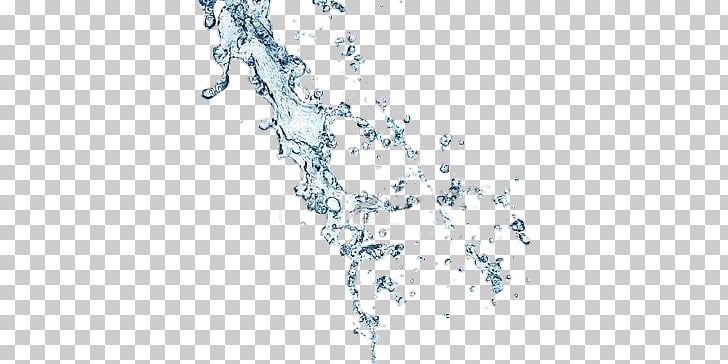The image depicts a dynamic stream of bluish-white water pouring from the top left to the bottom right over a background of small, meticulously arranged white and light gray checkered squares. The pattern, reminiscent of a tablecloth, spans at least 15 horizontal rows and over 20 vertical columns. The water, with its silvery and light blue tint, cascades down at a 45-degree angle, creating a sense of motion and chaos. Tiny droplets and bubbles scatter around the main stream, enhancing its volatile and un-uniform appearance. The entire scene is framed within a horizontal rectangle that is approximately twice as wide as it is tall, emphasizing the expansive spread of the watery splash against the geometric precision of the checkered backdrop.